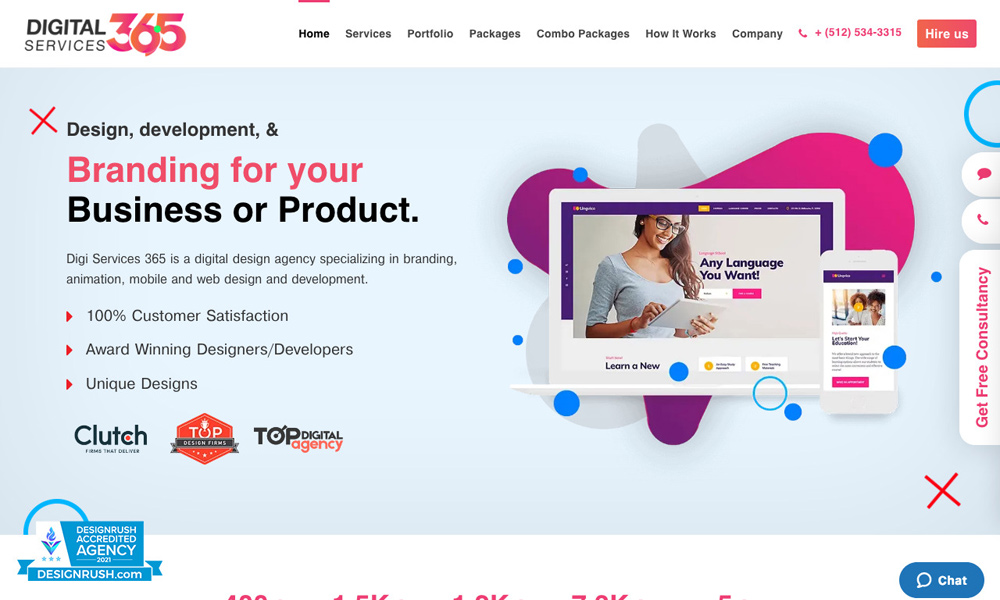The homepage of the website "Digital Service 365" prominently displays its name with "365" highlighted in pink, while the rest of the text is in black. Navigation options are arranged across the top, including Home, Services, Portfolio Packages, Combo Packages, How It Works, and Company. A phone number is prominently displayed in pink, alongside a "Hire Us" button in a pink box. The Home tab has an indicative pink line above it.

Beneath the navigation bar, a light blue box features the text: "Design, Development, and Branding for Your Business or Product." To the left, a pink X marks the section introducing Digi Services 365 as a digital design agency that excels in branding, animation, mobile, and web design and development. The agency boasts a 100% customer satisfaction rate, highlighted with pink arrow bullet points that emphasize:
- Award-winning designers and developers
- Unique designs

The site is endorsed by partnerships with Clutch, Top Digital Agency, and another unidentified top organization. Below this section, the text "Design Brush, Accredited Agency" is accompanied by the website URL "designbrush.com."

An image showcases a woman with brown hair and glasses, typing on her computer. The scene is set against an appealing background of pink, purple, gray, and blue dots, featuring a caption that reads: "Any Language You Want." On the right side, an adjacent section features a phone displaying the same advertisement and a call-to-action, "Get Free Consultancy," also highlighted in pink.